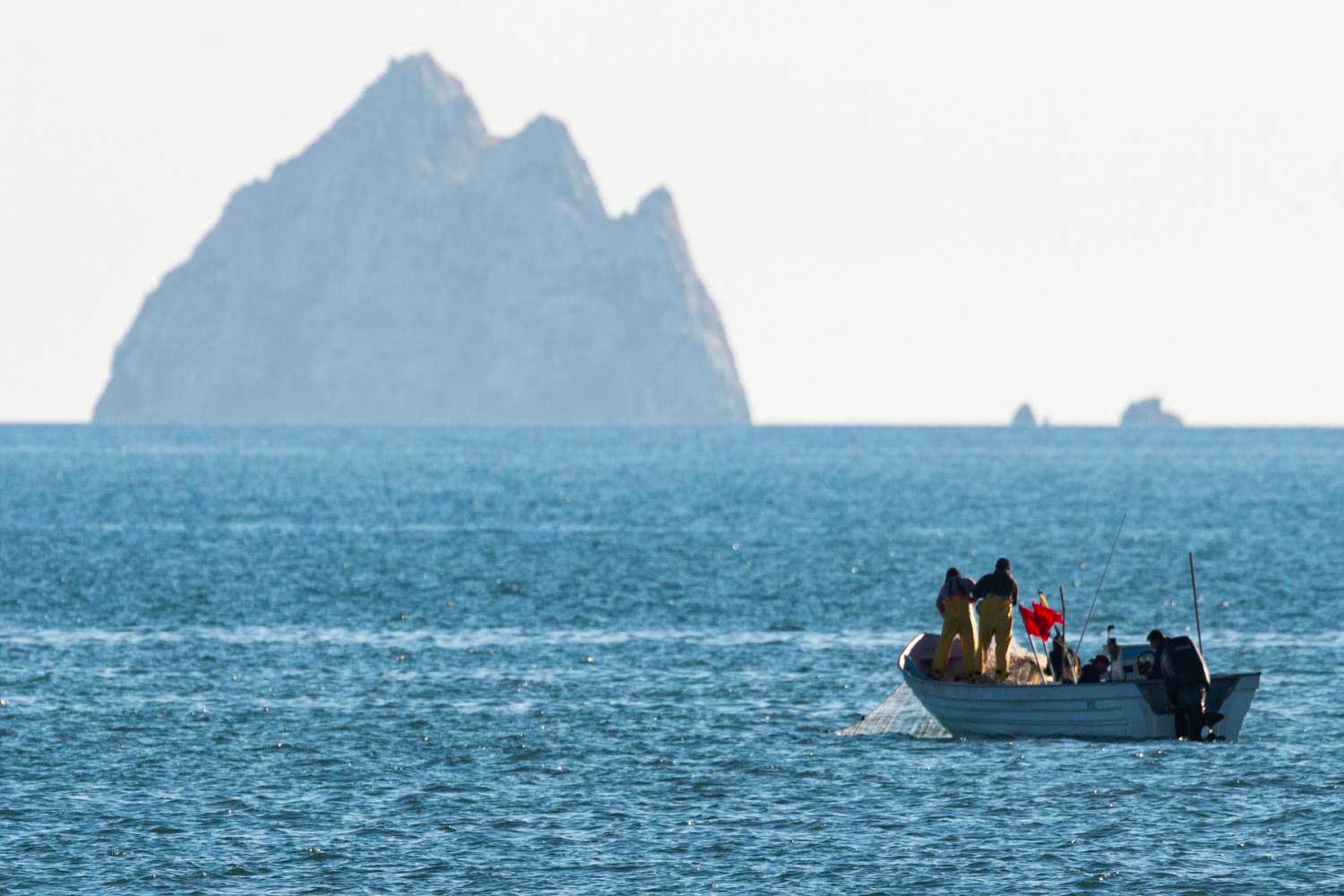In this photograph, a small white fishing boat with a red fabric trim is navigating the vast, open seas. The focus is on two men clad in yellow overalls, typical fishermen gear, who are standing aboard the boat, pulling up a large net from the water. There is also a fishing rod hanging off the side of the vessel. One man seems to be controlling the boat, while another person, perhaps a third member of the crew, is seen to the side. Red flags are visible on the boat. The surrounding water is vividly blue, with intricate details captured. In the far background, a hazy horizon reveals several rocky mountainous islands, with one appearing closer than the others. The sky has a slight haze, adding to the overall serene yet industrious atmosphere.